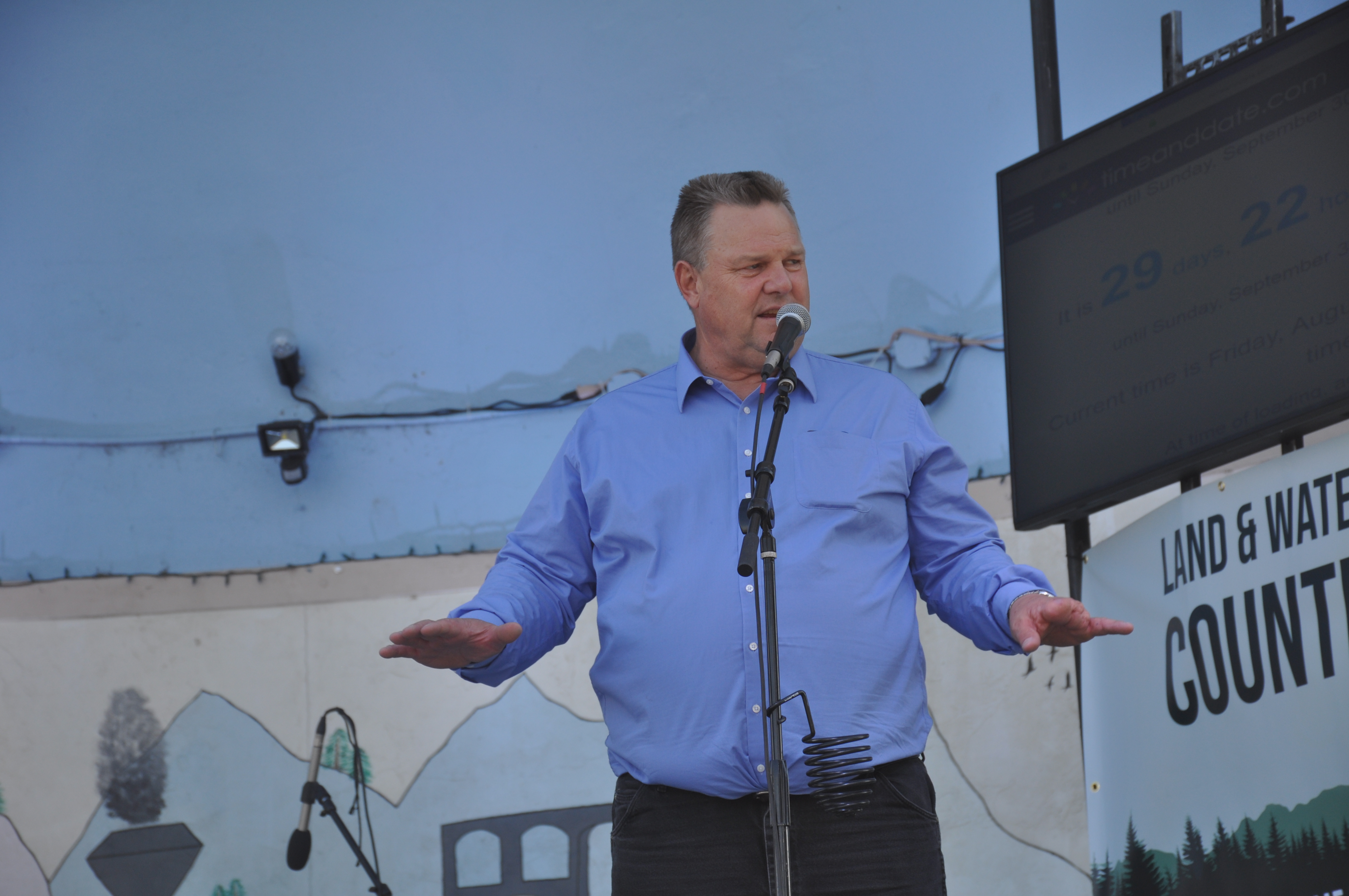This image depicts a man in the midst of delivering a speech. He stands at a microphone stand with the microphone positioned directly in front of his face. He has grayish-black hair and is dressed in a long-sleeved blue collared shirt, paired with either gray or blue jeans. His two hands are extended in front of him.

The setting is likely indoors, although there are some elements that might suggest an outdoor environment. Behind him, there is a sign with blue numbers "29" and "22" and a partially readable text that says "land and water count". Below this, the sign features simple designs of green mountains and evergreen trees, all set against a white background.

The background also includes a blue wall adorned with a string of lights and additional unclear wiring and lighting elements. Some unidentifiable graphics are present on this wall, contributing to the overall decor. An additional microphone is seen to the speaker's left, which he is not using. Despite some ambiguity, the dominant blue hues and the partial visibility of various elements add to the busy yet purposeful atmosphere of the scene.